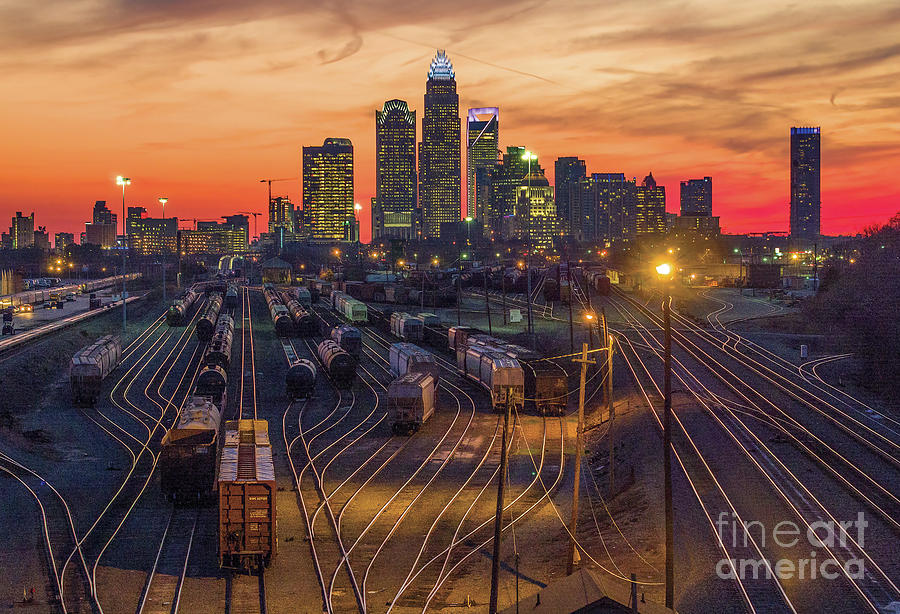This image, a digitally generated panoramic photograph in landscape orientation, showcases a vibrant city skyline at dusk. The sky is an intriguing mix of golden, orange, and red hues at the horizon, gradually darkening to a grayish tone with swirly dark clouds above. The city is adorned with a variety of tall buildings and skyscrapers, the tallest at the center featuring a striking blue light structure. All buildings are illuminated, their windows glowing with yellow light, indicating it's evening and transitioning to nighttime, as evidenced by the active streetlights.

In the foreground, the image captures a complex railway yard with an array of rail lines in both straight and spiral patterns. Multiple rail cars and train carts are seen on the tracks, some static while others appear to be in motion. The photograph shows three different perspectives of the scene, stitched together to form a wide strip format: a left view with shorter structures, a central view dominated by the tallest skyscrapers, and a right view featuring medium-height buildings with converging tracks but no rail cars.

Adding authenticity, the bottom right corner of the image carries the watermark "Fine Art America." The image exemplifies photographic representationalism and realism, emphasizing the dynamic and intricate details of a city at dusk juxtaposed against the busy railway yard below.